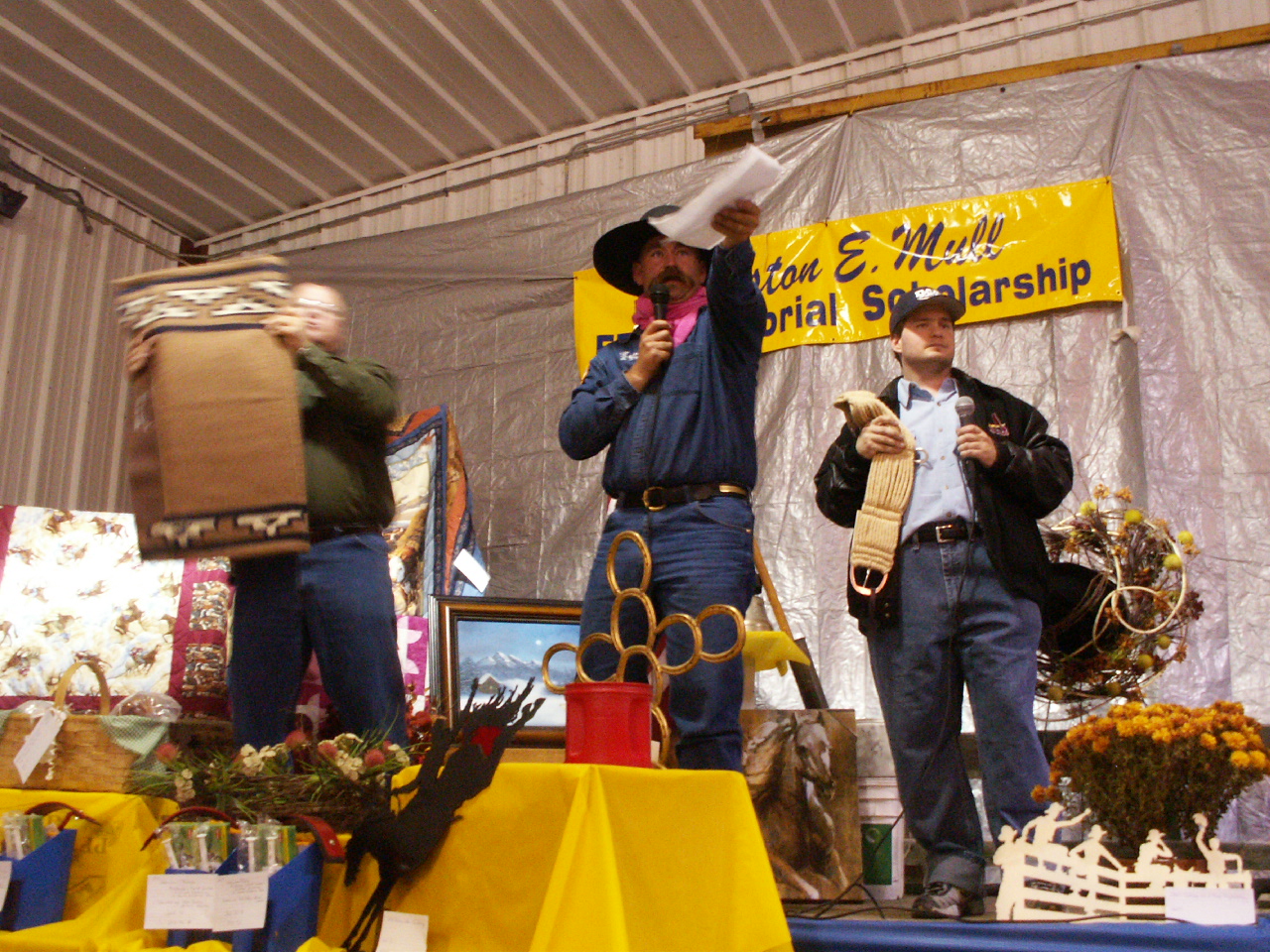In this vibrant and bustling indoor scene, three men stand prominently on a stage adorned with numerous eclectic items ranging from flowers and pots to rings and rugs, hinting at an auction event. The man at the center, presumably the auctioneer, sports a cowboy hat, a red bandana around his neck, a blue shirt, and blue pants. He is holding a microphone in one hand and pointing towards the crowd with the other, emphasizing his role in directing the event. To his right, another man in blue jeans, a light blue collared shirt, a dark jacket, and a black baseball cap stands, grasping a belt. To the left, a third man wearing blue jeans and a brownish shirt holds up a tan rug decorated with white, pyramid-shaped designs. They are framed against a backdrop comprising a vinyl covering with a partially visible yellow banner reading “E. Mullen Scholarship” in blue letters, and silver slats crisscrossing the light white roof above. The stage itself is blue, with knee-high tables draped in yellow cloths and surrounded by an array of flowers, adding to the lively ambiance of the gathering.